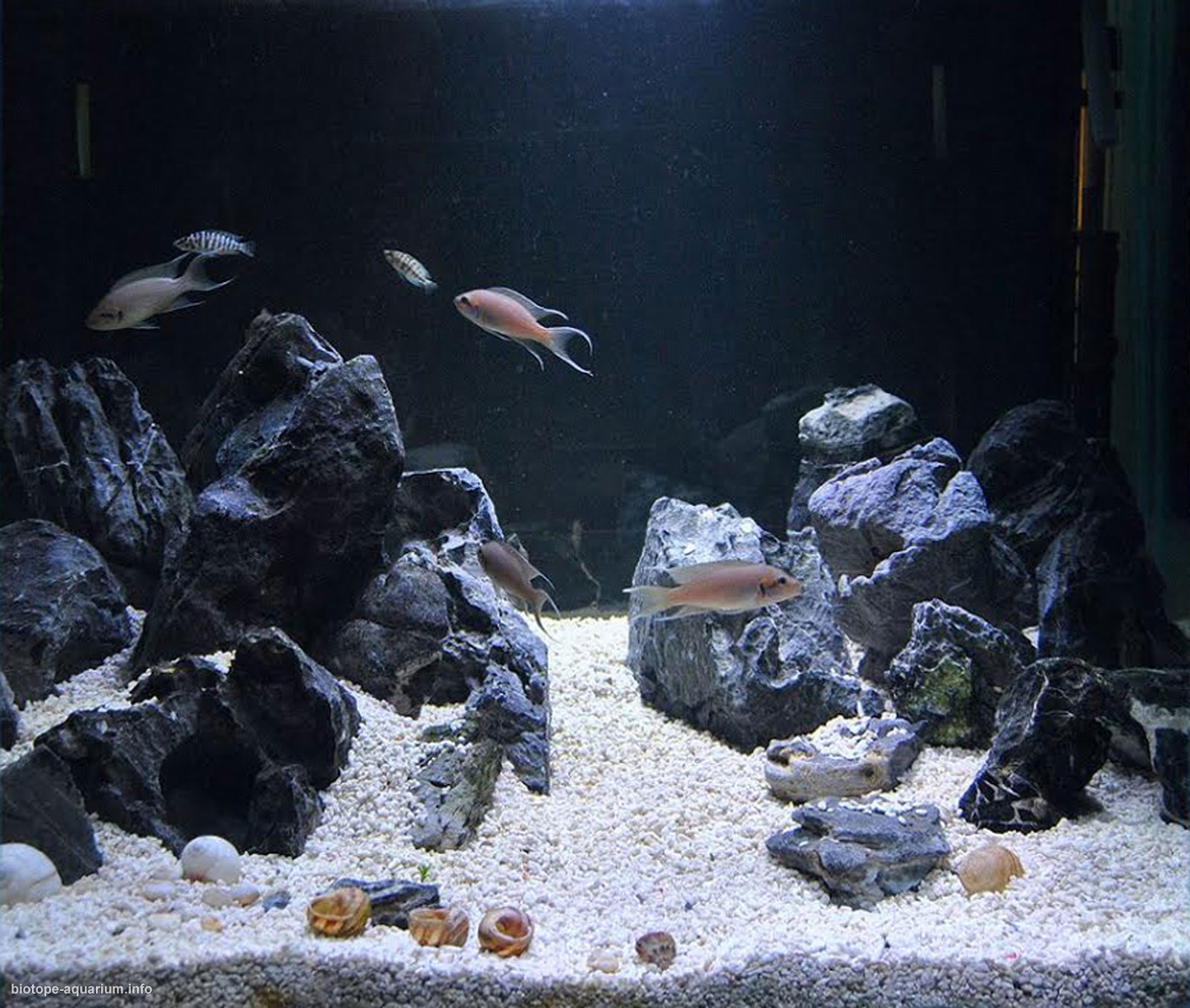The photograph showcases a dark-themed aquarium with a black background, prominently lit by a single white light from the top, highlighting the aquatic life within. The base of the tank is covered with small white gravel, interspersed with larger stones and a variety of shells—some white and others beige or brown. The rocks are primarily black and gray, contributing to the tank's natural aesthetic. There are a total of seven fish in the tank. Among them, four medium-sized fish exhibit a light salmon-pink color, while two smaller fish display distinct zebra stripes. Additionally, there is one smaller, off-white, opaque fish. The glow from the top light diffuses through the water, making the vividly colored fish clearly visible against the stark, dark backdrop. The bottom left corner of the image bears the text "biotopeaquarium.info."